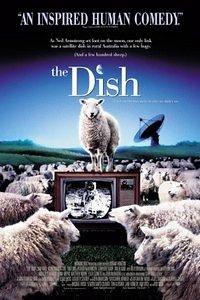The movie poster for "The Dish" portrays a whimsical and satirical scene set in a vast green grassy field teeming with sheep. At the center is an old, retro brown television set displaying a fuzzy black-and-white image of an astronaut, a nod to the first moon landing. Sitting atop this TV is a single sheep with white wool, gazing directly at the viewer. Surrounding the television are dozens of sheep, all seemingly engrossed in the broadcast as they stretch into the rolling green hills in the distance. To the right side of the poster, near the middle of the image, the shadow of a large satellite dish points toward the top left, suggesting a connection to the TV's broadcast. The sky transitions from blue to deep purple and black near the top of the image, providing a dramatic backdrop. Dominating the upper portion of the poster, a bold white quote reads "An inspired human comedy," subtly hinting at the film's satirical nature. Just beneath this quote, the title "The Dish" is prominently displayed, with the dot on the "i" cleverly represented by a moon, encapsulating the movie’s whimsical and reflective tone.